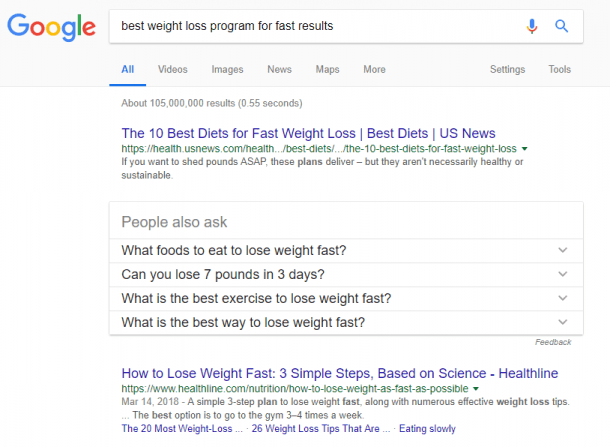This is an image of a Google search results page. At the top, in the search bar, the query "best weight loss program for fast results" is entered, accompanied by the Google logo on the left, which is depicted in its iconic blue, red, yellow, and green colors. The search yields approximately 105 million results in 0.55 seconds.

The first search result is titled "The 10 Best Diets for Fast Weight Loss" from the U.S. News & World Report at help.usnews.com. The snippet highlights that these plans can help shed pounds quickly, but they may not necessarily be healthy or sustainable in the long term.

Additionally, there is a "People also ask" section with questions such as "What food to eat to lose weight fast?", "Can you lose 7 pounds in 3 days?", "What is the best exercise to lose weight fast?", and "What is the best way to lose weight fast?".

The search result below is from Healthline, titled "How to Lose Weight Fast: 3 Simple Steps, Based on Science" located at helpline.com/nutrition/how-to-lose-weight-as-fast-as-possible. It mentions offering a simple 3-step plan to lose weight quickly.